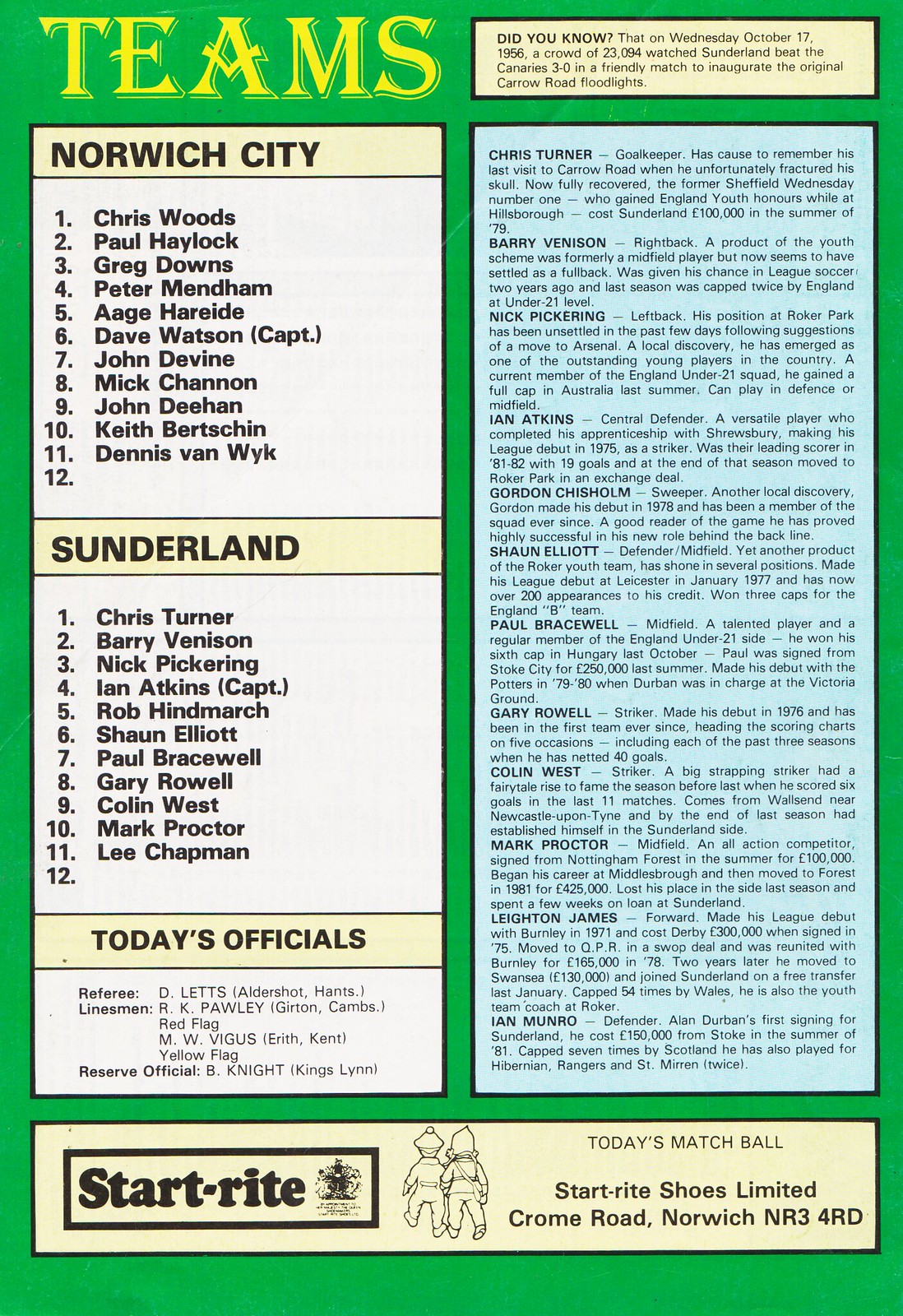The image depicts a vibrant sports flyer predominantly featuring a St. Patrick's Day green background. At the top left, the word "Teams" is prominently displayed in a yellow font. Below this title, two football teams are listed: Norwich City and Sunderland, each with their respective player line-ups numbered from 1 to 11. Further down, the flyer names the match officials, including referee D. Letts, with assistants R. K. Pauly, W. V. Vigas, and reserve official B. Knight.

On the right-hand side of the flyer, a small rectangular box at the top includes a historical trivia caption reading: "Did you know? On Wednesday, October 17, 1956, a crowd of 23,094 watched Sunderland beat the Canaries 3-0 in a friendly match to inaugurate the original Carrow Road floodlights." Directly below this, inside a blue rectangle that occupies most of the right side, is detailed information about the players' names and positions, including notable mentions such as Chris Turner, Barry Venison, Nick Pickering, Ian Atkins, and Mark Proctor.

At the bottom, a rectangle spans the width and notes the sponsor of the event: "Start Right Shoes Limited, Chrome Road, Norwich, NR3, 4RD" in black text.